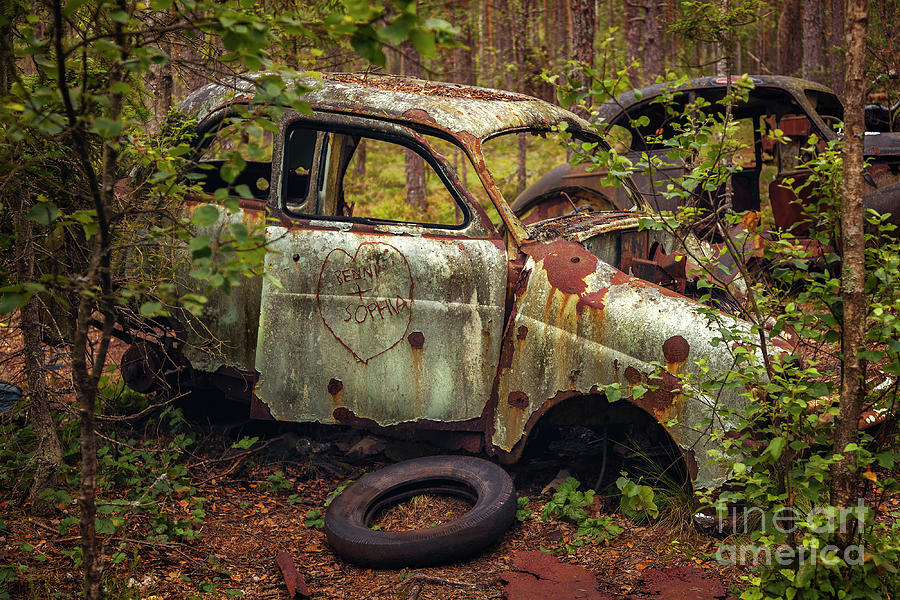This detailed photograph captures an evocatively decaying, European-style car from the 1950s, abandoned in a wooded clearing. The central car, a grayish-green relic, sits prominently with its rusted and graffiti-marked passenger door partially open, displaying the names "Ben + Sophia" inside a heart. The vehicle, heavily rusted and perforated with bullet holes, is missing its hood, revealing an exposed engine, and lies stripped of its tires except for a solitary rubber tire on the ground before it. Tangled within the faded splendor of the forest, characterized by vibrant summer or spring foliage, a dark, partially concealed second car from the same era can be glimpsed, obscurred by shrubbery and blending into the tree trunks, it too, forlorn and decaying. Both vehicles suggest a story of abandonment and time’s relentless reclamation, all underscored by the subtle "Fine Art Media" inscription in light lime lettering at the bottom right of the image.